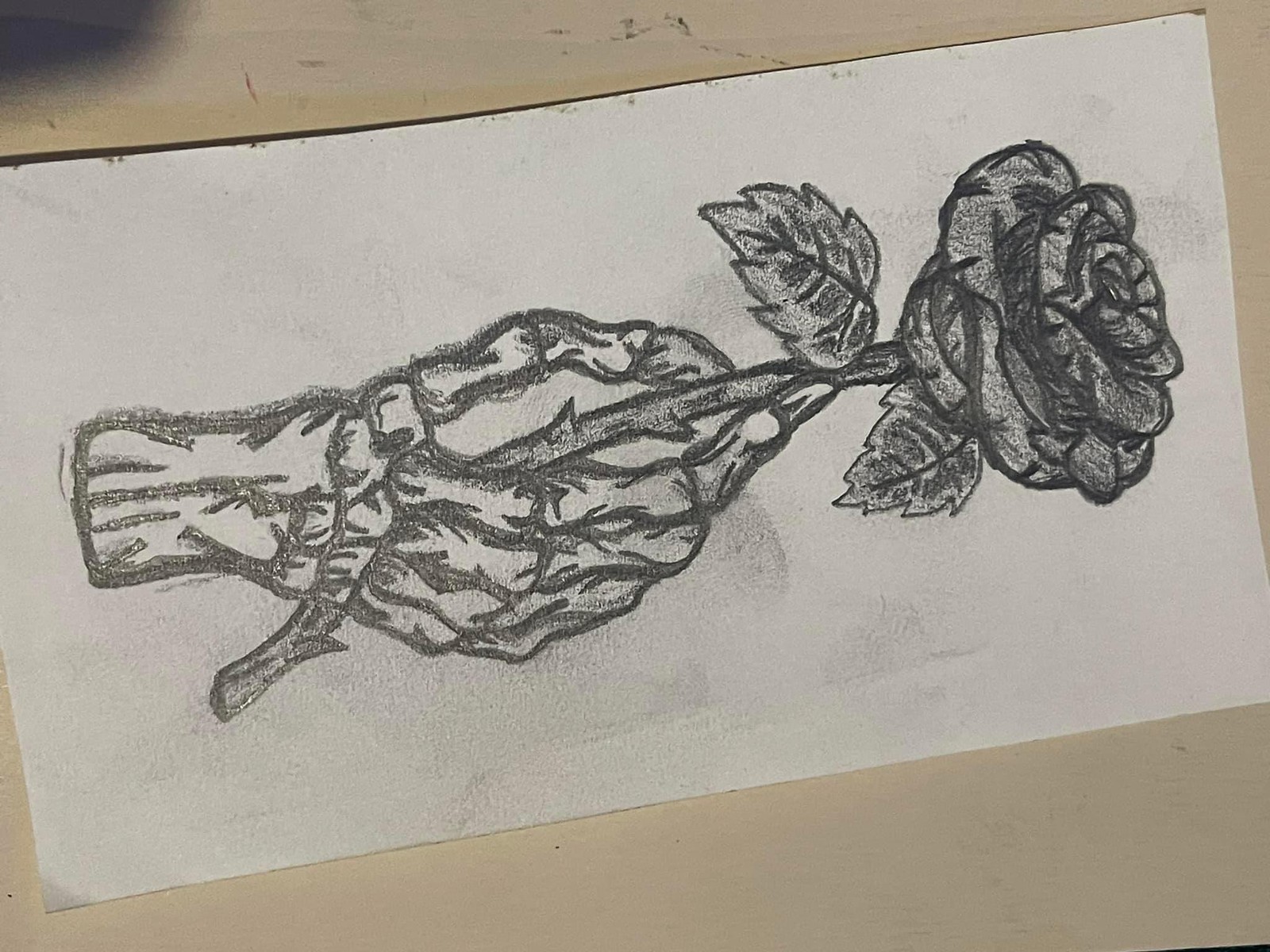This is a photograph of a pencil-sketched, black-and-white drawing on a rectangular piece of white paper, which is larger than a standard sheet. The sketch is placed on a white or light cream-colored piece of furniture, possibly a table or an easel, and the image is oriented horizontally. The drawing features a skeletal hand gripping a long-stemmed rose with visible thorns. The rose is fully bloomed, with two detailed leaves at the base of the bud, one on each side. The sketch employs dark, thick lines for the outlines and abstract, exaggerated shading to emphasize wrinkles in the hand and the details of the rose petals, creating a contrast with lighter pencil shading on the leaves and petals. There are also noticeable charcoal smudges on the paper, adding to the sketch's textured appearance.